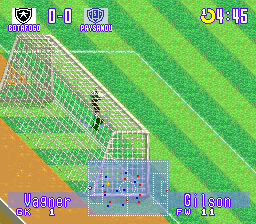In this video game scene, a lush field is depicted with alternating dark green and light green stripes, creating a visually appealing contrast. A large net is prominently positioned at one end of the field, with a goalie stationed in front of it, indicating an imminent soccer match. The names "Bada Fago" and "Prasamu" are displayed at the top of the screen, while "Wagner" and "Gilson" appear at the bottom, along with the respective abbreviations "GK1" (goalkeeper) and "FW" (forward) beside each name, defining their in-game roles. Notably, there is a small sandy spot situated behind the goalie, adding a touch of realism to the scene. Additionally, a blue target is visible in the center bottom of the screen, possibly indicating a strategic point or a target for gameplay. The scene is set with a timestamp of 4:45, suggesting a specific moment in the match.